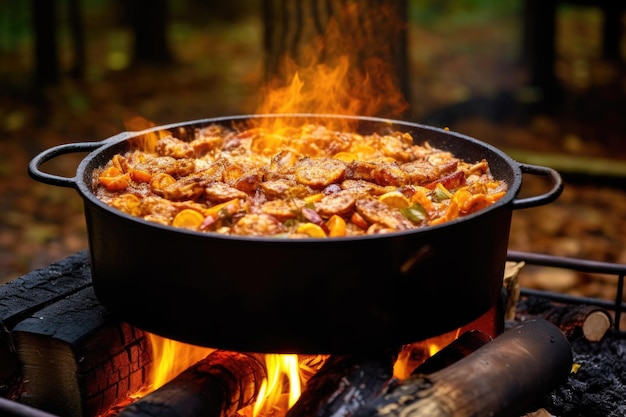This image depicts a horizontally aligned rectangular scene of a large, cast iron pot with handles on each side, positioned on an outdoor grill with visible flames and burning logs underneath. Inside the pot, there appears to be a stew or casserole comprising of round slices of sausage and possibly orange peppers, bathed in a yellowish mix. The flames underneath are intense enough to emerge through the sides of the pot, giving an impression of the food being engulfed by the fire. In the backdrop, the scene is set in a wooded area with blurred views of tree trunks and green foliage, hinting at a forest environment. Metal bars can be seen behind the pot, likely part of the burner setup. The overall atmosphere suggests an outdoor cooking scenario, possibly in the early morning or early evening as hinted by the dim yet present light, with the focal point clearly on the sizzling meal within the pot.